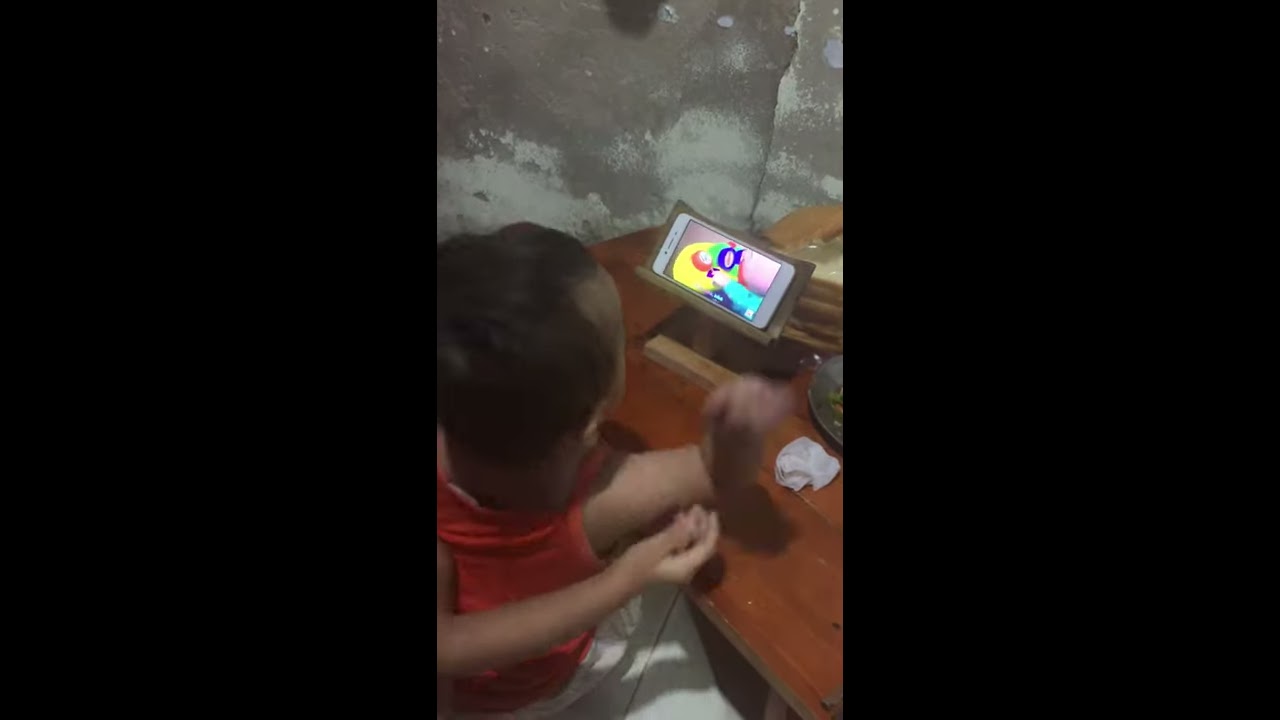This photograph, taken in portrait orientation, captures a young child seated on a cement floor, intently watching a cartoon on a mobile phone mounted on a wooden bench. The child, dressed in a red shirt, sits in the center of the image, their right arm resting on the table. The room has gray, unpainted walls with white patches. The scene is framed by black borders on the left and right sides, emphasizing the child as the focal point. The child's light brown skin and dark brown hair are illuminated by the colorful figures on the phone's display, which include hues of yellow, orange, purple, and pink, along with light blue. Another child, only partially visible, has an arm around the seated child, suggesting a protective or supportive gesture.